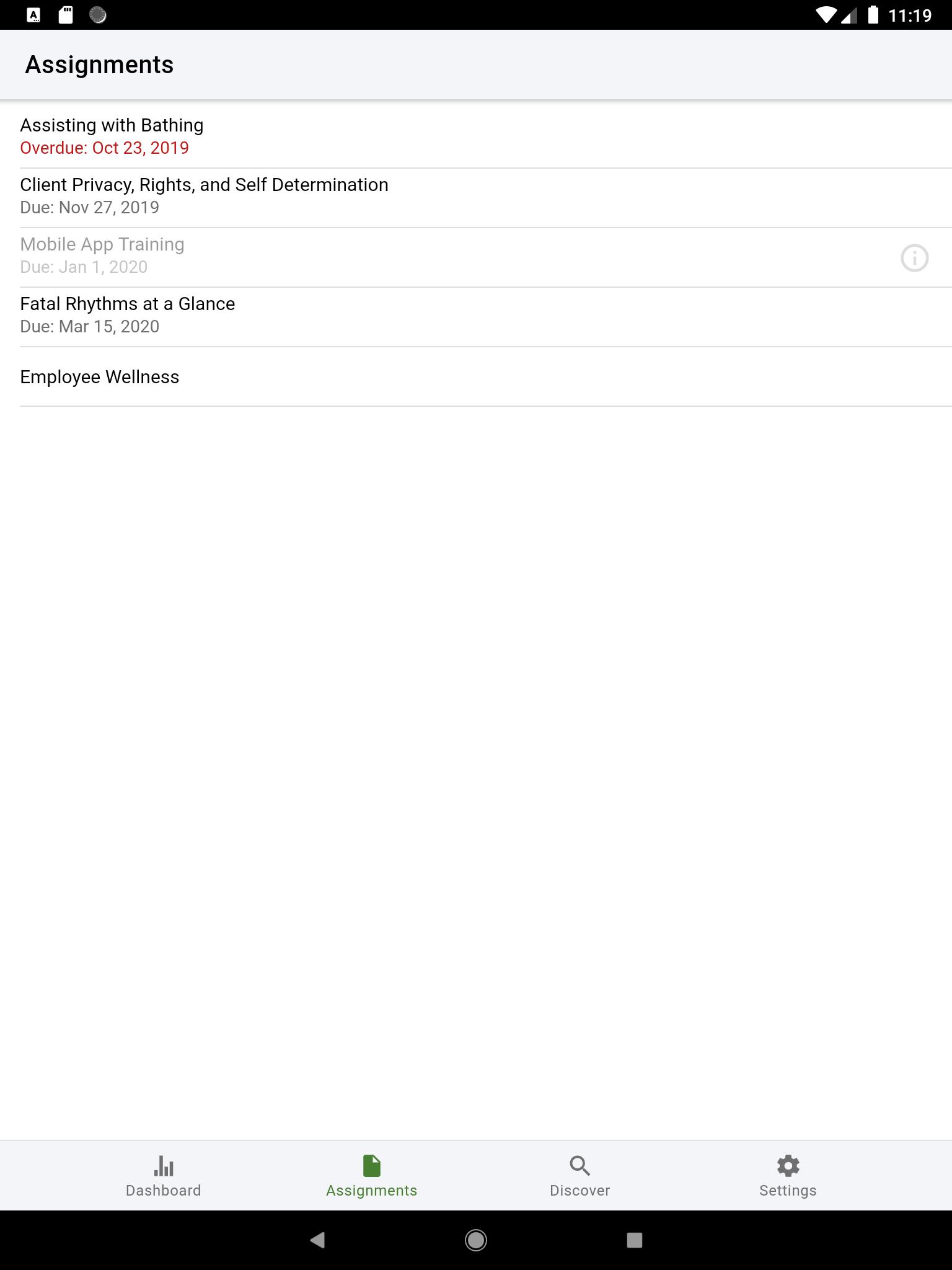The image depicts a structured display of assignments and due dates, organized within a digital interface. 

At the very top, there is a horizontal black bar functioning as a header, housing various small icons on both its left and right sides. Beneath this bar, the word "Assignments" is prominently displayed in bold black font, followed by a thin light gray line.

Under this, in standard black font, is the text "Assisting with bathing," immediately followed by the word "Overdue" in red font, with the due date "Oct 23, 2019" in the same red color. Another thin gray line separates this from the subsequent section.

Next, in regular black font, appears the text "Client Privacy Rights and Self-Determination," with the due date "Nov 27, 2019" in gray font below it. Another horizontal thin gray line demarcates this from the following section.

The text "Mobile App Training" is displayed in light gray font next, with "Due: Jan 1, 2020" beneath it. This is followed by another thin gray line.

Further down, in black font, it reads "Fatal Rhythms at a Glance," with "Due: Mar 15, 2020" displayed below in light gray font. This section is followed by another thin gray line.

Then, in black font, the text "Employee Wellness" appears, accompanied by another thin gray line below it. The rest of the page transitions into blank space until the bottom.

At the bottom, there are two horizontal rectangular areas. The first is light gray, centrally featuring the text "Dashboard" in light gray font with an icon above it. Adjacent to it is a green area marked "Assignments," which includes a green icon. The rest of the bar goes back to light gray with "Discover" accompanied by a magnifying glass icon, and "Settings" alongside a gear icon.

Below all of this, a black area with simple geometric icons is visible, including a triangle pointing left, a circle, and a square.